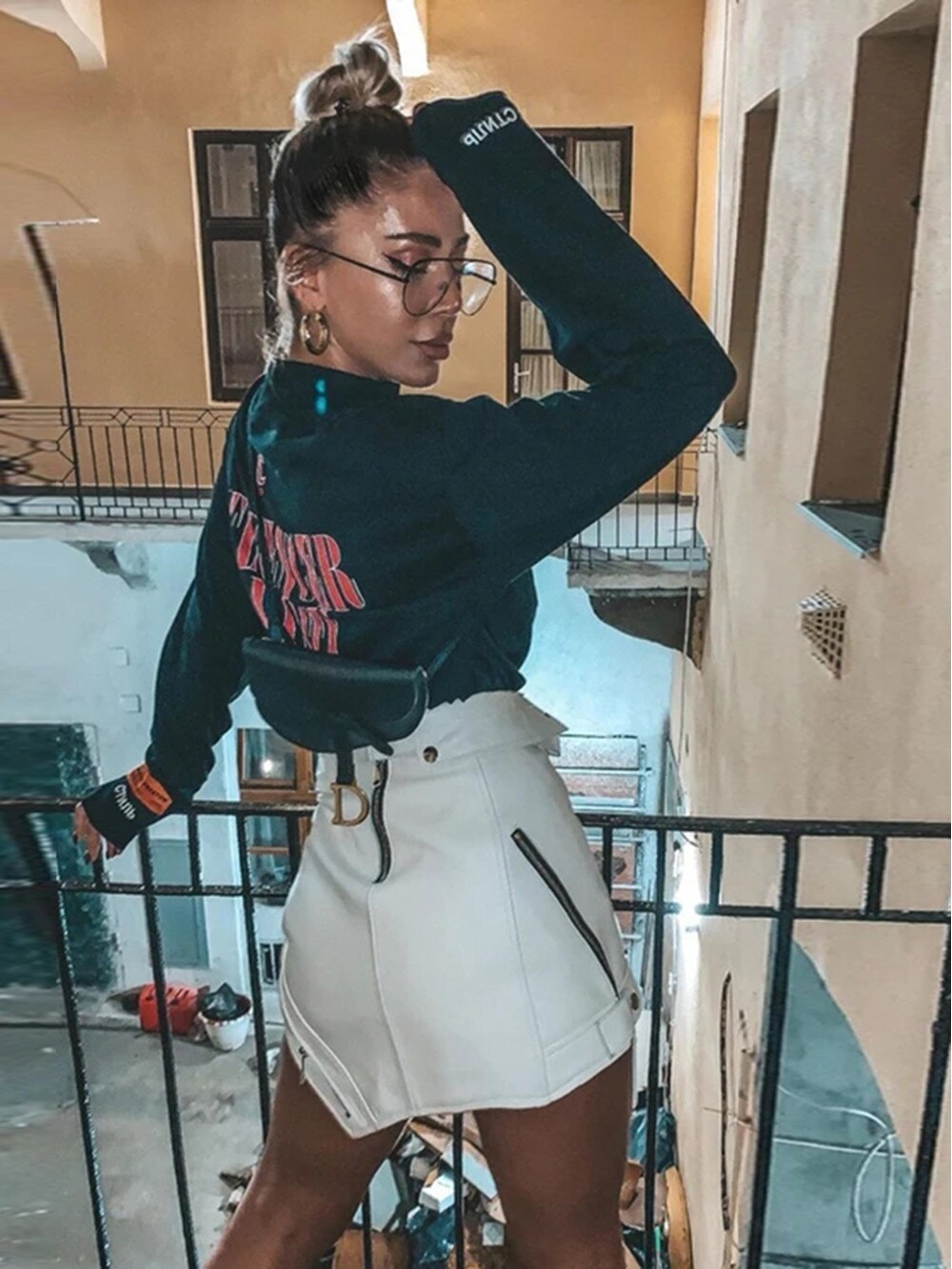A young woman, possibly a model, stands on the second floor of an apartment building against a black metal railing. Her body is facing away, but her head is turned back towards the camera, offering a clear view of her face, accented by round glasses and gold hoop earrings. She has dark brown hair pulled up into a ponytail, and she wears a black long-sleeved top with white letters "C-T-N-U-B" above the wrists and red writing on the back, though it is difficult to read due to wrinkles. One arm is raised, with her fist resting on her forehead, giving her a pensive look. Her other hand rests on the black metal barrier. She sports a very short black leather mini skirt adorned with zippers and black outlines. Her legs are tan, possibly indicating a dark-skinned tone or a deep tan. A black pouch slung around her shoulder hangs off her back. Behind her, the backdrop includes light brown walls with window frame openings, another black barrier in the distance, and a contrasting light blue-colored lower wall. The street below is cluttered with items like pails and a gas can, adding to the urban atmosphere of the scene.